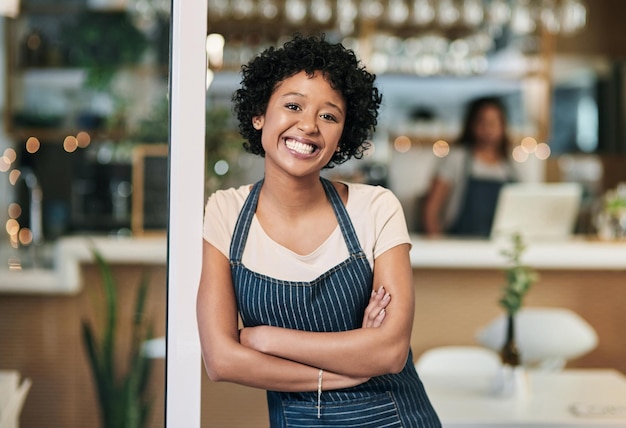In the photograph, a vibrant, beautiful woman stands proudly in the foreground, leaning casually against a sliding door frame with her arms crossed. She has radiant, toned skin and loose, curly afro hair, which frames her beaming smile. Dressed in a crisp white t-shirt, she is adorned with a stylish, pinstriped denim apron, and a delicate bracelet dangles from her wrist, adding a touch of elegance. Her appearance suggests she might be of mixed race, possibly of African descent, and her joyful expression exudes confidence and warmth.

The background, which is intentionally blurred, hints at a lively bar or café setting. Here, you can discern tables, a well-lit bar area, and design elements that add to the restaurant's welcoming atmosphere, such as a colleague in the same uniform who appears to be engaged with a computer screen. The scene is illuminated with natural brightness, enhanced by twinkling reflections that resemble tiny orbs of light scattered throughout the image. A plant placed on the floor adds a touch of greenery and completes the inviting ambiance. The photograph captures not only the setting but also the essence of the subject’s pride and happiness in her work, making it feel both professional and heartwarming.